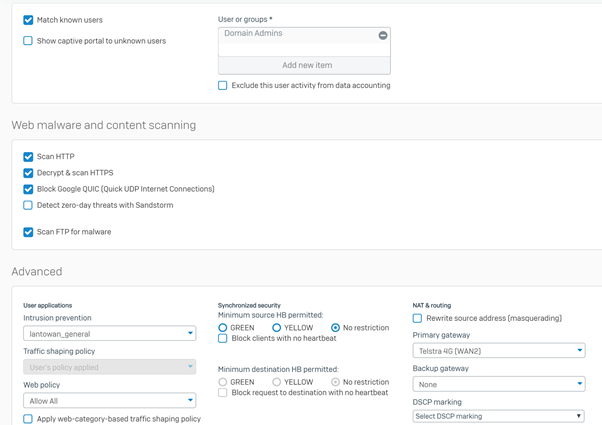### Screenshot Overview

The screenshot is divided into three distinct sections, each enclosed within a white box. Here’s a detailed breakdown of each section:

#### First Section:
- **Untitled Section:**
  - Contains two checkboxes on the left-hand side:
    - **Match known users:** This checkbox is selected and highlighted in blue.
    - **Show captive portal to unknown users:** This checkbox is not selected.
  - To the right:
    - A smaller box labeled **User Groups** includes an entry for **Domain Admins**.
    - At the bottom of this box, there's an option labeled **Add new item** centered within the box.
  - Below this:
    - Another checkbox labeled **Exclude this user activity from data accounting** remains unchecked.

#### Second Section:
- **Titled: Web, Malware, and Content Scanning:**
  - Contains a white box below the title with several options:
    - Four items within this white box are checked.
    - The fourth item, **Detect zero-day threats with Sandstorm**, is not checked.

#### Third Section:
- **Titled: Advanced:**
  - Divided into three subsections:
    - **User Applications:** 
      - Includes various options with a checkbox at the bottom labeled **Apply web category-based traffic shaping policy,** which is not checked.
    - **Synchronized Security:**
      - Includes multiple configurations but no specific details about checkboxes or options.
    - **NAT and Routing:**
      - Features a checkbox labeled **Rewrite source addresses,** which is located directly underneath the NAT and Routing title, and this checkbox is selected.

This screenshot captures a comprehensive view of various settings and options available, from user matching and activity exclusion to advanced traffic and security configurations.